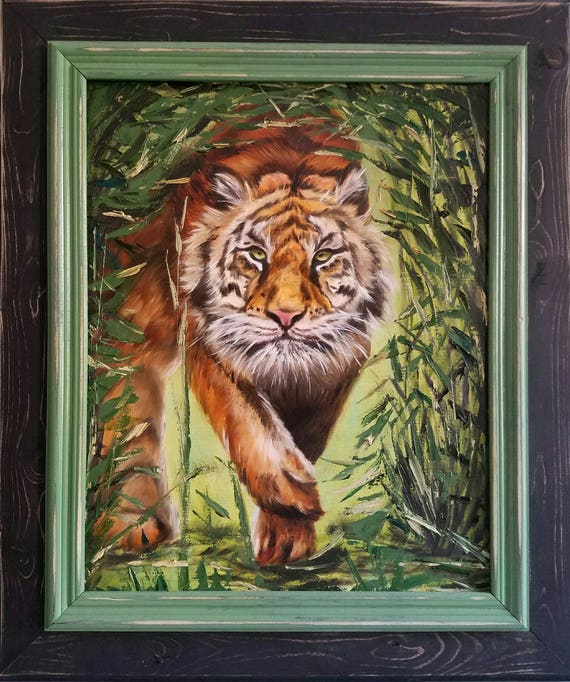This semi-realistic painting depicts a majestic tiger stealthily emerging from a tunnel of lush green foliage, eyes fixed intently forward. The tiger's striking orange fur with black stripes, white accents around the mouth, and light green eyes create a vivid contrast against the vibrant greenery. The attentive feline is portrayed in a low, forward-crouching stance, giving the impression it is sneaking up or advancing towards the viewer. Its right paw is slightly lifted, poised in mid-air, while the left paw firmly touches the ground. Various shades of green from the surrounding grass blades and foliage enhance the depth and movement within the scene. The painting is beautifully framed with a double-layer design: an inner medium-tone green wooden frame that complements the greenery in the artwork, encased by a thicker outer frame of dark, almost black wood with rich textures and natural knots. The overall composition, from the intricate details in the tiger’s fur and eyes to the dynamic, luminous foliage, offers a breathtaking glimpse into the wild's raw and captivating beauty.